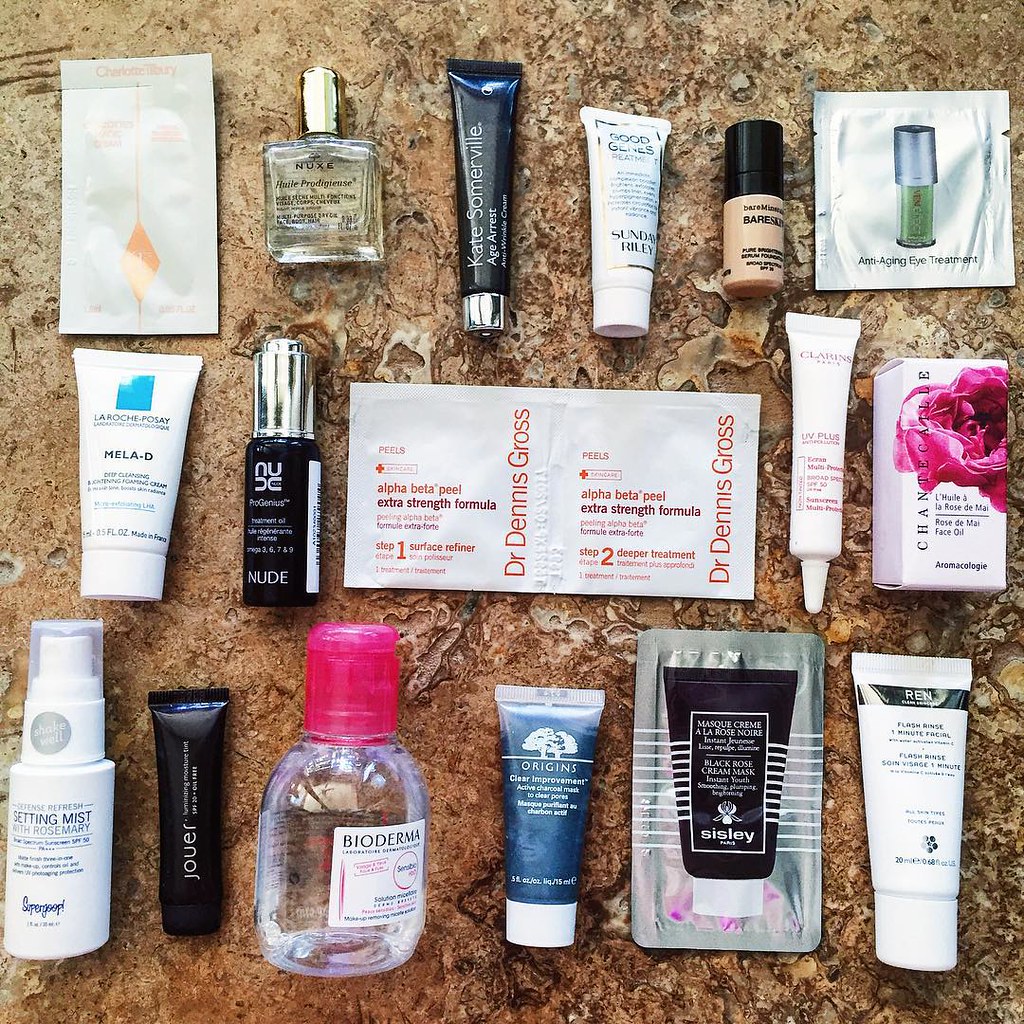The image showcases an assortment of around 15 makeup products and skincare items, all set against a predominantly brown background that appears to be either a piece of wood or a digital representation. The background includes hues of brown and white, creating a rustic yet clean aesthetic. 

Central to the image is a white packet prominently labeled "Dr. Dennis Gross Alpha Beta Peel Extra Strength Formula" in red and purple lettering. Surrounding this key item are various products, including:

- A clear Bioderma bottle with a pink top.
- A blue tube of Origins, presumably an ointment.
- A black Jouer container located at the bottom left.
- A silver packet from Sisley positioned at the bottom left.
- A white packet featuring a green and silver illustration.
- A "Setting Mist" spray in a white bottle.

The items vary in color, including black, silver, white, cream, green, and pink, providing a visually diverse array of cosmetic and skincare essentials.